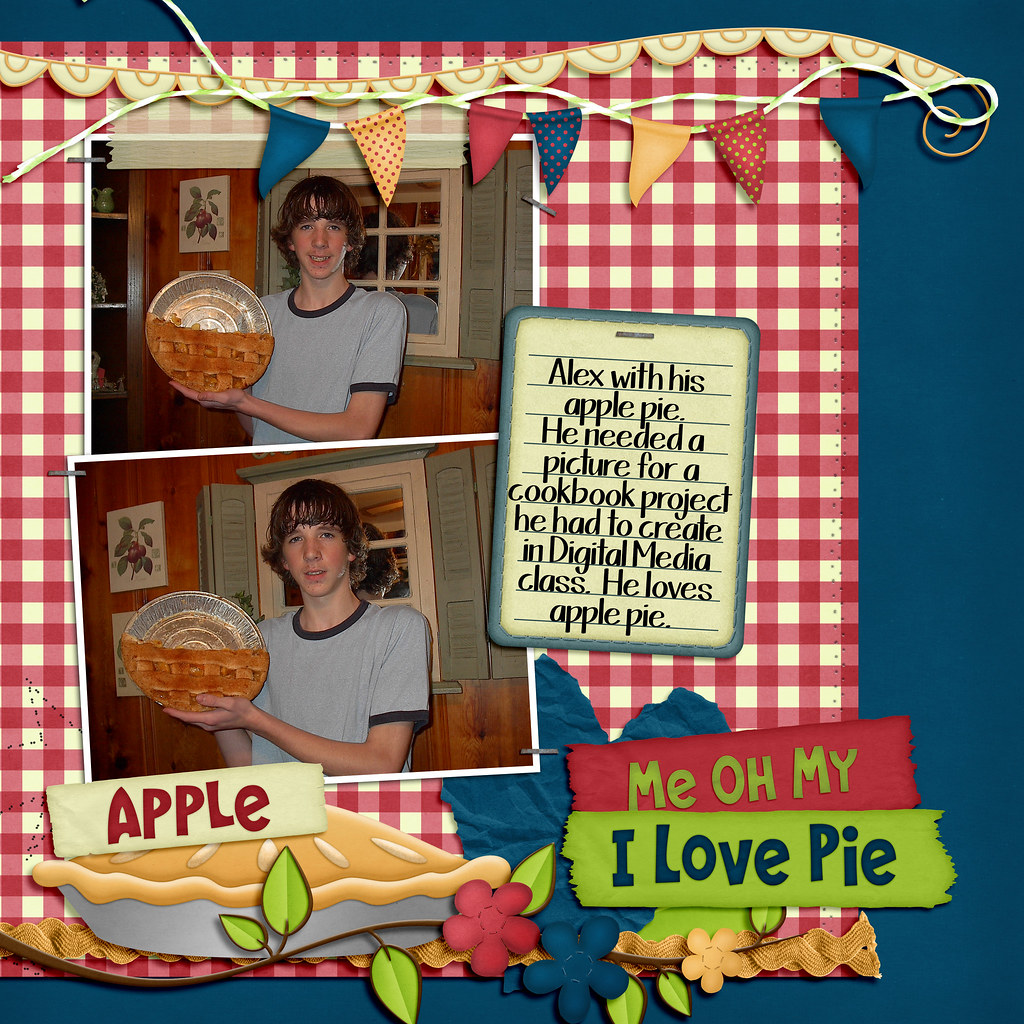The image is designed to resemble a page from a scrapbook, set against a red and white gingham-patterned background. It features two photographs of a young boy named Alex, each showing him holding a half-eaten apple pie on a silver pie plate, with the latticework on the remaining pie clearly visible. Alex, who has brown hair falling over his eyes, is wearing a blue t-shirt with matching blue collar and sleeves, and is smiling at the camera in both images. Behind Alex, there is a wall with gray shutters and a window, and in one version of the description, there are cabinets and some drawings on the wall, while reflections in the glass window can also be seen.

The colorful decorations include a series of small pennants in blue, yellow, and red hanging down towards the photographs and some ribbon along with decorative text that reads "Alex with his apple pie; he needed a picture for the cookbook project he had to create in digital media class." Additional embellishments include stickers and clip art of an apple pie with the word "apple" in red script, and a whimsical caption in green letters on a red background that says "me oh my," followed by "I love apple pie" on a green background. The design also features decorative flowers and leaves, emphasizing the scrapbook theme. The caption notes that Alex loves apple pie and that the image was part of a digital media class project.